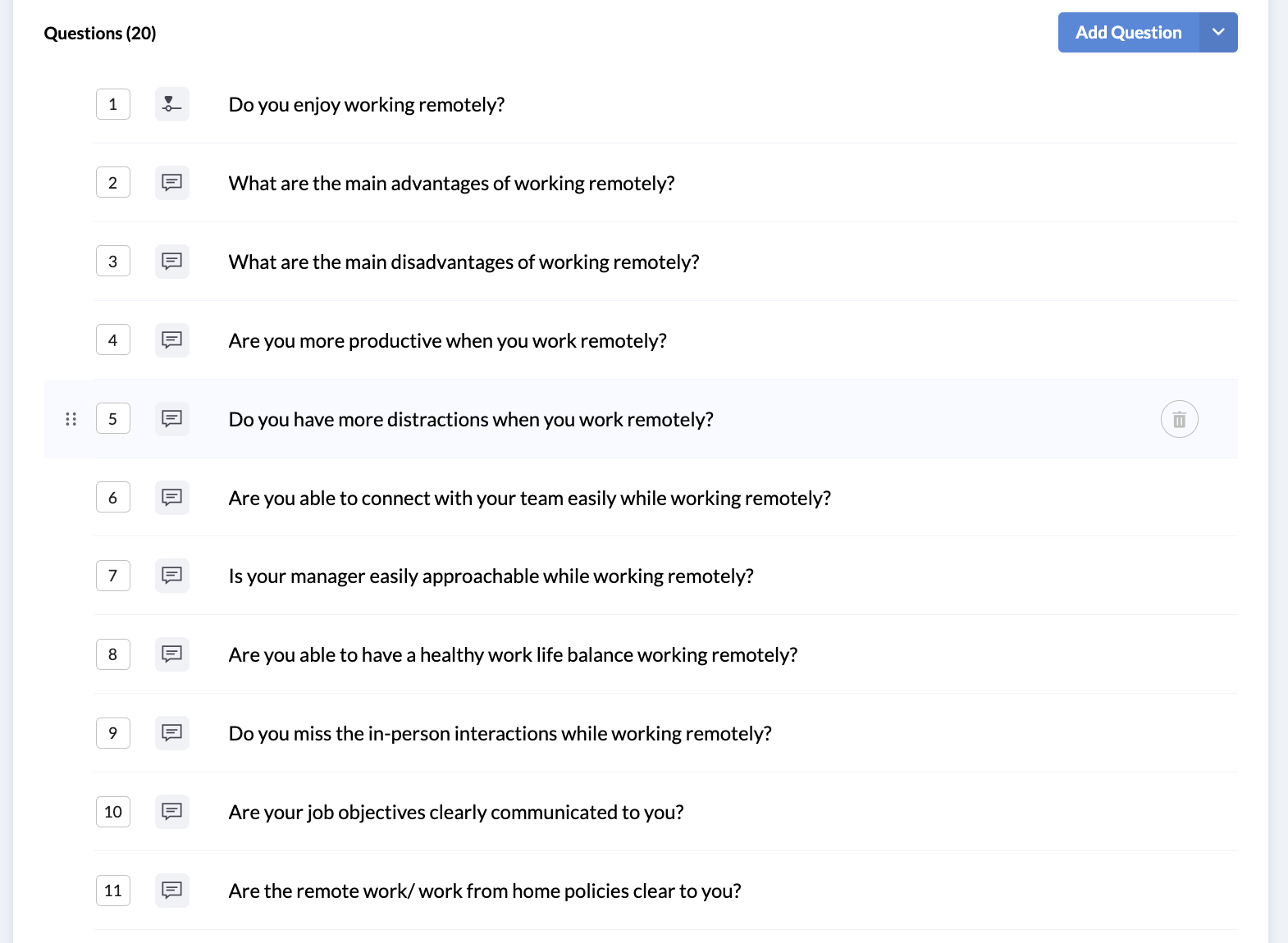This image displays a list titled "Questions (20)" in black letters at the top left corner. To the right of this title, there is a blue button labeled "Add Question," accompanied by an arrow suggesting a dropdown menu. Currently, the list shows 11 questions, each with a speech or chat bubble icon between the question number and the text, except for the first question which features a heart over a bar icon instead. All question numbers are enclosed in squares, with the fifth question highlighted in a darker gray color. 

The questions listed are:
1. Do you enjoy working remotely?
2. What are the main advantages of working remotely?
3. What are the main disadvantages of working remotely?
4. Are you more productive when you work remotely?
5. Do you have more distractions when you work remotely?
6. Are you able to connect with your team easily while working remotely?
7. Is your manager easily approachable while working remotely?
8. Are you able to have a healthy work-life balance while working remotely?
9. Do you miss in-person interactions while working remotely?
10. Are your job objectives clearly communicated to you?
11. Are the remote/work from home policies clear to you?